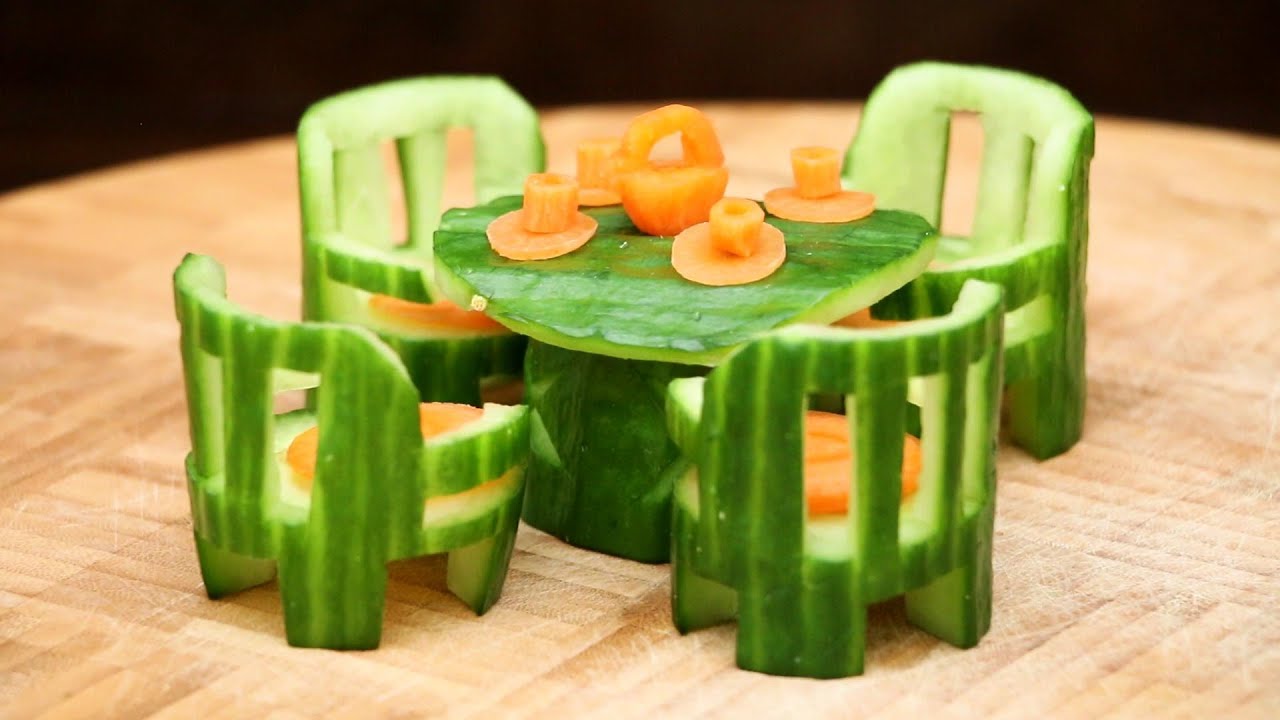This is a detailed color photograph showcasing an intricate piece of food art set against a black background. The centerpiece of the image is a meticulously crafted table and four chairs, all made from carved cucumber skins. The table, composed of a green pedestal and a matching green tabletop, stands on a brown checkered or butcher block wood surface. Surrounding the table are four cucumber chairs, each complete with slatted backs and armrests, carved seamlessly out of single pieces of cucumber. 

Enhancing the vivid display, each chair features an orange carrot slice serving as a cushion, creating a striking contrast. Atop the table, also crafted from carrot, are four cups and four saucers, arranged as if for a tea party. Centrally placed on the table is an orange basket, adding a final touch to this colorful and whimsical arrangement. The entire scene is set on a surface that appears to be light tan, suggesting either wicker or wood, adding to the natural feel of the composition.